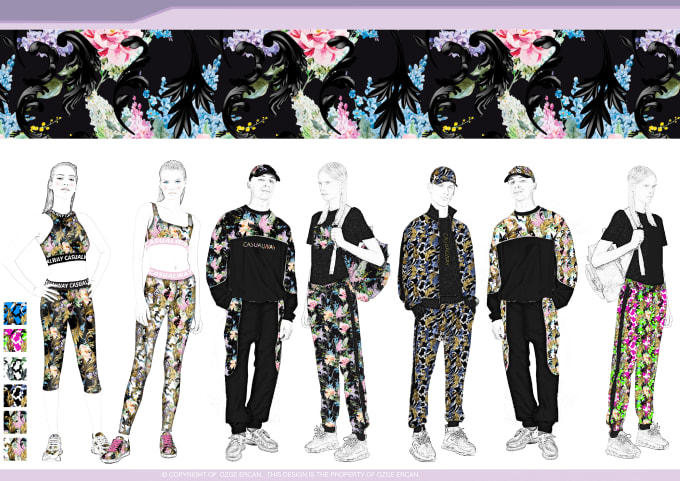This rectangular illustration, likely from a fashion catalog or website, features a detailed representation of trendy teen apparel. Across the top of the image is a long, angled tab reminiscent of a manila folder tab, rendered in light lavender against a darker lavender background. Below this tab is a striking horizontal band that stretches from left to right, adorned with a vivid tropical floral design. This design includes stylized black swirls resembling acanthus leaves, lush tropical foliage, and vibrant floral elements such as spikes of pink and white flowers, accompanied by clusters of blue flowers, contributing to an intense tropical ambiance.

Beneath this decorative band, the background transitions to white, displaying pencil sketches of seven teenagers modeling various outfits. On the lower left side of the image, there are six small square swatches showcasing different patterns, including the one seen in the broad top band. Each swatch appears to be clickable, suggesting that selecting a swatch magnifies the corresponding pattern across the top band for enhanced visibility.

The seven sketched figures are as follows:

1. **Female Teenager:** She has her hands on her hips, wearing a halter top and cropped leggings that extend below her knees.
2. **Female Teenager:** Attired in a bralette-style top paired with long leggings.
3. **Male Teenager:** Donning a baseball cap and a sweatsuit comprising a black pullover top and black bottoms, accentuated with floral pattern trim along the chest, arms, and down each side of the legs.
4. **Female Teenager (Left Profile):** With her hair styled in pigtail braids, she sports a backpack, a short-sleeved black t-shirt, and sweatpants, all featuring the floral pattern.
5. **Male Teenager:** Wearing an open jacket and matching pants in either a camo or floral pattern, complemented by a ball cap in the same design.
6. **Male Teenager:** Similar to the third figure, he wears a pullover sweatshirt and sweatpants with black top and bottom, distinguished by a different pattern.
7. **Female Teenager (Right Profile):** Mirroring the previous outfit, she dons pants with a different vibrant pattern, a black t-shirt, and a plain sketch-based backpack without color.

All these outfits incorporate various dynamic patterns, demonstrating a range of stylish and colorful options for trendy teen apparel.